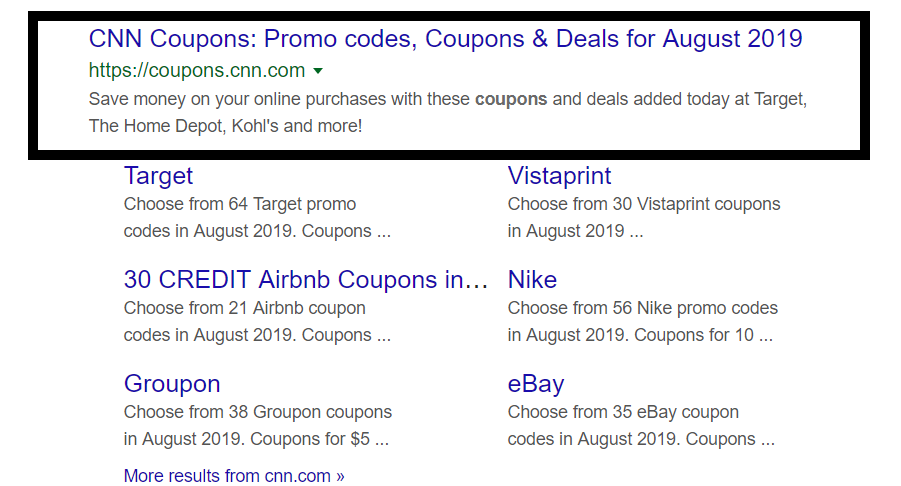The image showcases a webpage featuring various clickable links, seven in total, each styled with a blue font for the titles and black font for the descriptions. The top link is distinctly highlighted by a long black rectangle and reads, "CNN Coupons, Promo Codes, Coupons and Deals for August 2019, coupons.cnn.com." Below this primary link, there are six additional options: one from Target, one from Groupon, one from eBay, one from Nike, one from Vistaprint, and one labeled "30 Credit Airbnb Coupons." The overall design features an all-white background, with each of the links standing out in blue and black text. In the bottom left corner of the page, another blue link reads, "More Results from CNN.com," indicating an option for further navigation.